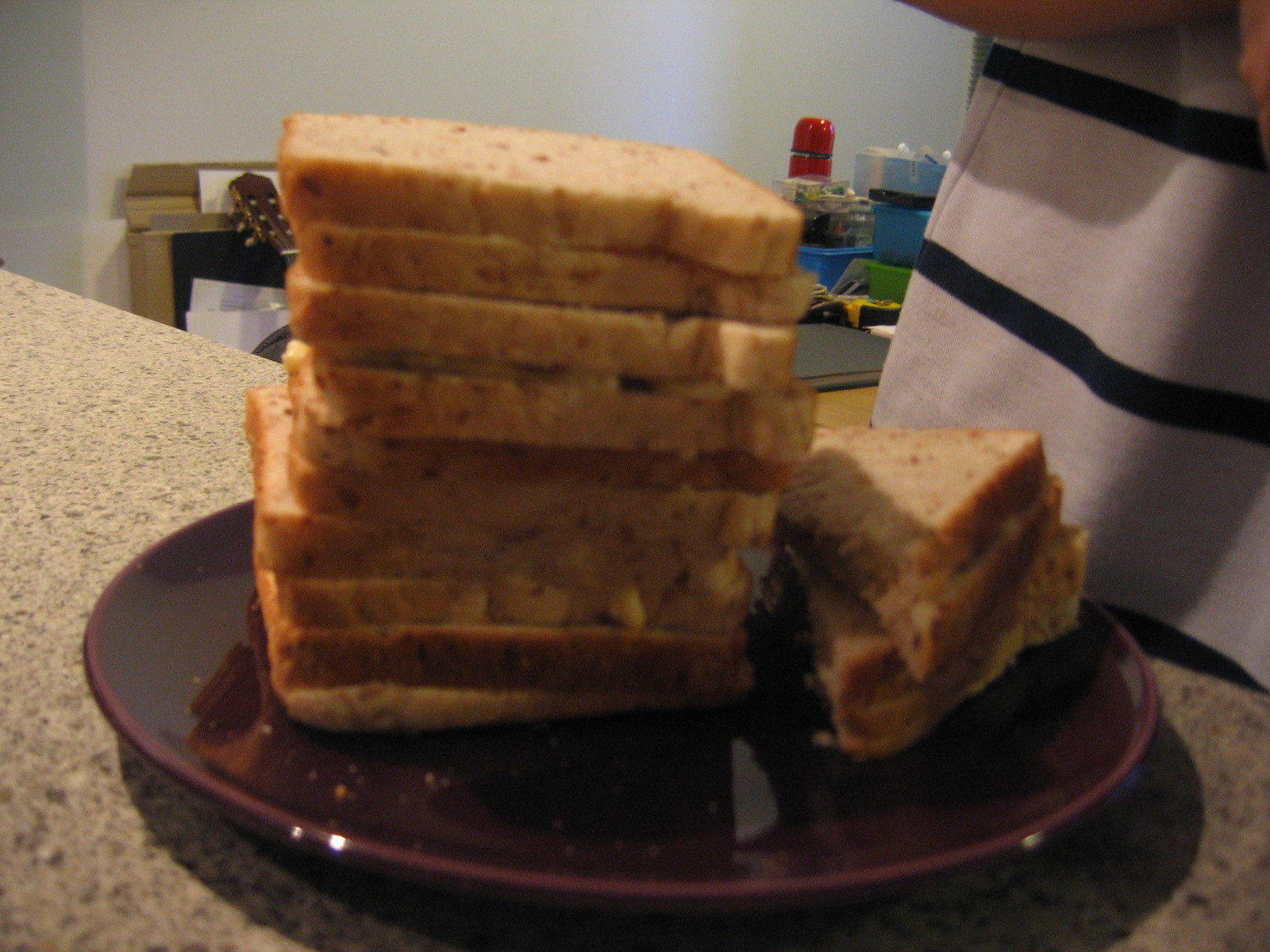In a slightly cluttered kitchen, a deep burgundy, glossy ceramic plate sits atop a light tan and speckled granite countertop. On the plate, a stack of approximately ten slices of thinly sliced, multi-grain wheat bread is arranged, with hints of a beige filling—possibly peanut butter—occasionally peeking through. To the right of the stack, a sandwich cut diagonally into two triangular halves is neatly stacked. Behind the plate, a person wearing a white shirt with navy blue stripes stands. Their presence partially obscures a small shelf filled with assorted items, including a red thermos, blue bins, and what appear to be random kitchen items. The neck of a guitar leans against the shelf, adding a unique touch to the scene. The overall atmosphere is one of a cozy yet slightly cluttered kitchen, captured in moderate lighting and a somewhat blurry photo.